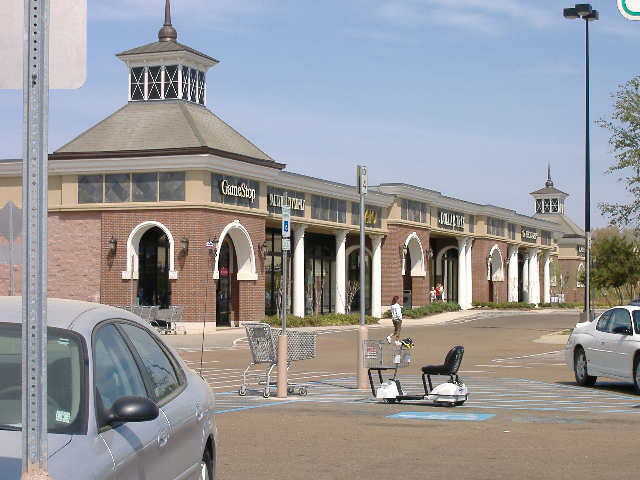The photograph captures a vibrant strip mall set against a clear, sunny day. The architectural design of the strip mall is particularly striking, featuring red brick facades accented by elegant white archways and columns between the storefronts. Above, a sloping roof culminates in a stylish peak reminiscent of the Twin Spires at the Kentucky Derby, adding a touch of distinctive charm to the mall.

In the foreground, the asphalt parking lot is partially occupied by a parked car and several scattered grocery carts, including one oddly paired with a chair. A person can be seen walking across the lot, and a white car is parked to the right. The strip mall houses several stores, the most legible of which is a GameStop. There appear to be five or six additional stores, though their names are not clearly discernible.

A family is also present in the scene, with a mother carrying a baby and a child trailing behind. The overall image evokes a sense of everyday community life in a pleasant, well-maintained commercial setting.